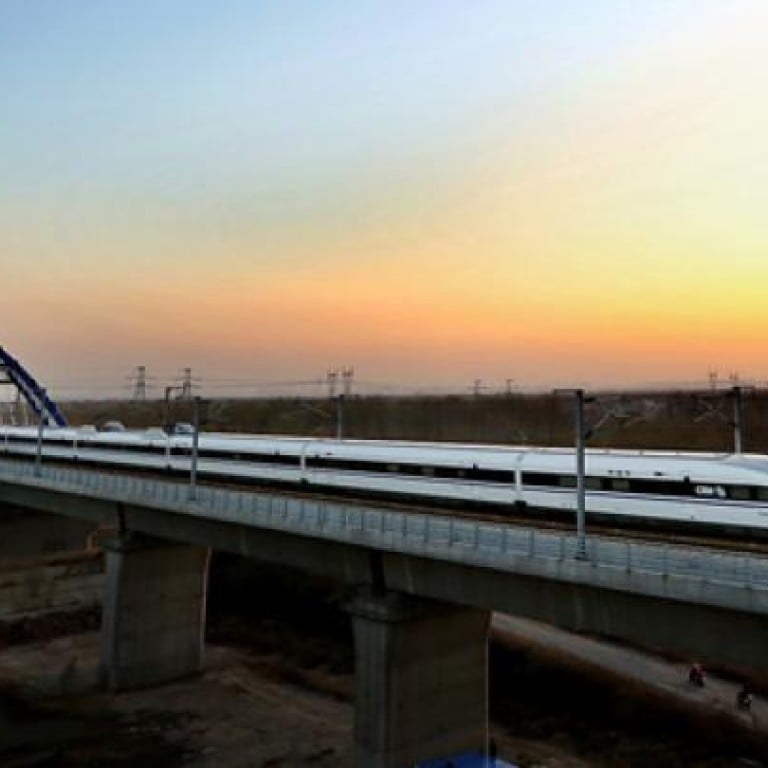The image captures a white monorail with black windows traveling from left to right on an elevated concrete track supported by two rectangular pillars. The track includes silver-colored horizontal rails and several utility poles with wires stretching across the scene. The landscape beneath the bridge is a mix of brown terrain and sparse vegetation. In the distance, there are indistinct, dark green trees and utility wires on tall metal poles. The sky above reveals a gradient of colors, starting with a light blue on the upper left, blending into pink, orange, and yellow hues towards the horizon, suggesting it is either sunrise or sunset. The overall atmosphere transitions from a serene twilight to the warmth of an incoming or receding daylight, with the brighter yellow tones concentrated on the right side of the image.